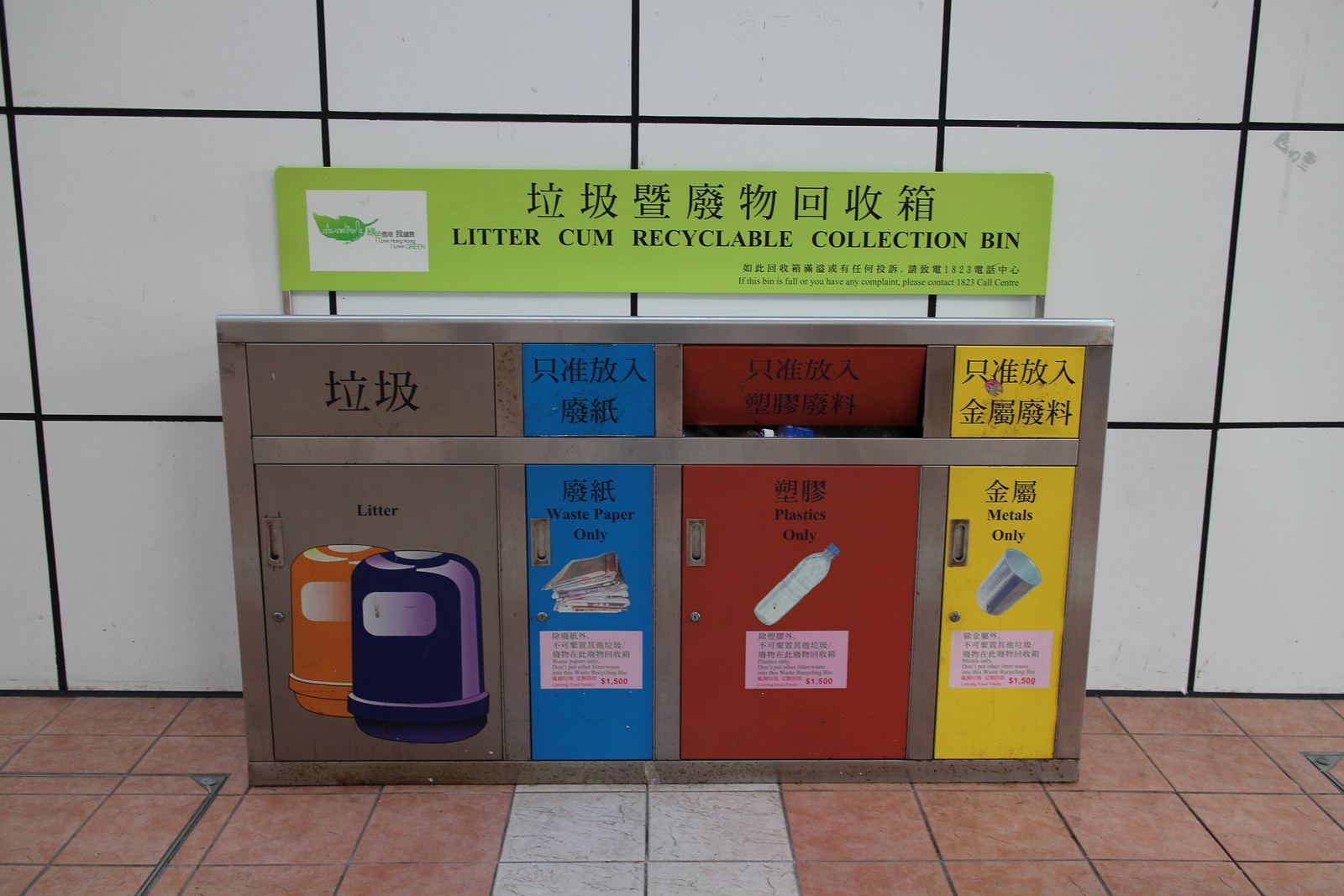The image features a stainless steel recyclable container bin with four distinct sections, positioned in front of a wall adorned with large white tiles and black grout. The floor is covered in a combination of predominantly orange-ish reddish-pink tiles interspersed with rows of white tiles. Above the bin, a green banner prominently displays the text "Litter-Cum-Recyclable Collection Bin" in both English and Japanese characters.

The bin itself is divided into four compartments: 

1. The first and largest section on the left is gray and labeled "Litter," although the accompanying illustration is somewhat ambiguous.
2. The second compartment is a narrower bright blue section labeled "Waste Paper Only," featuring an image of stacked paper.
3. Following this is a larger red compartment designated for "Plastics Only," marked with a picture of a water bottle.
4. The final and smallest section on the end is yellow, labeled "Metals Only," with an image of a metal cup.

The overall scene suggests an organized indoor recycling area clearly demarcated for different types of waste.